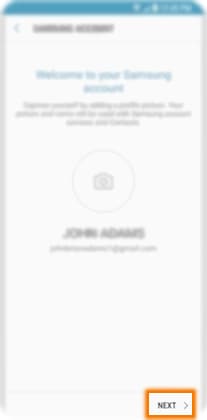A highly blurred and out-of-focus screenshot from a mobile device is depicted. Along the top of the screen is a thick teal-colored header, with indistinguishable white shapes in the upper right corner. The main body of the page has a white background. There seems to be a search box near the top, but it is too unclear to be certain. Below this, the page title, also in teal, is unreadable. The primary content appears to be a block of black text, possibly a description, though the specifics are obscured by the blurriness. In the center, there is an icon of a camera. Beneath the icon, what appears to be the name "John Adams" can be partially deciphered, followed by what is likely his email address. At the bottom right of the screen is a white button with an orange border, labeled "Next," accompanied by a right arrow, indicating a navigation function.